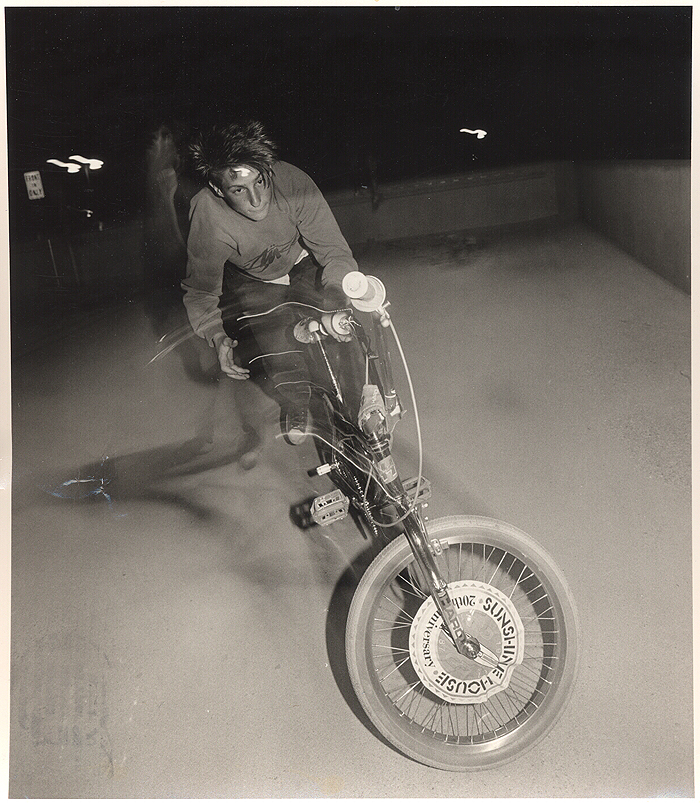In this black-and-white image, taken in a nighttime outdoor setting, the focus is on a young male who appears to be riding a modified bicycle or a homemade electric motor vehicle. The scene is centered on a cement or concrete surface, which could be a road or possibly a rooftop. The background is mostly dark, with faint, indistinct lights visible. There are no other visible objects or text in the image. The young man, dressed in a dark shirt, pants, and shoes, is sitting on the vehicle and holding onto its handlebars, with the front wheel slightly turned. The grayscale palette of the photo adds to the mystery and starkness of the image. The bicycle-like vehicle shows detailed wiring extending across the handlebars toward the seat, indicating a custom-built or modified design. The wheel is approximately 16 inches high, and the young man gazes towards the camera, though not directly at it, adding an element of candidness to the composition.